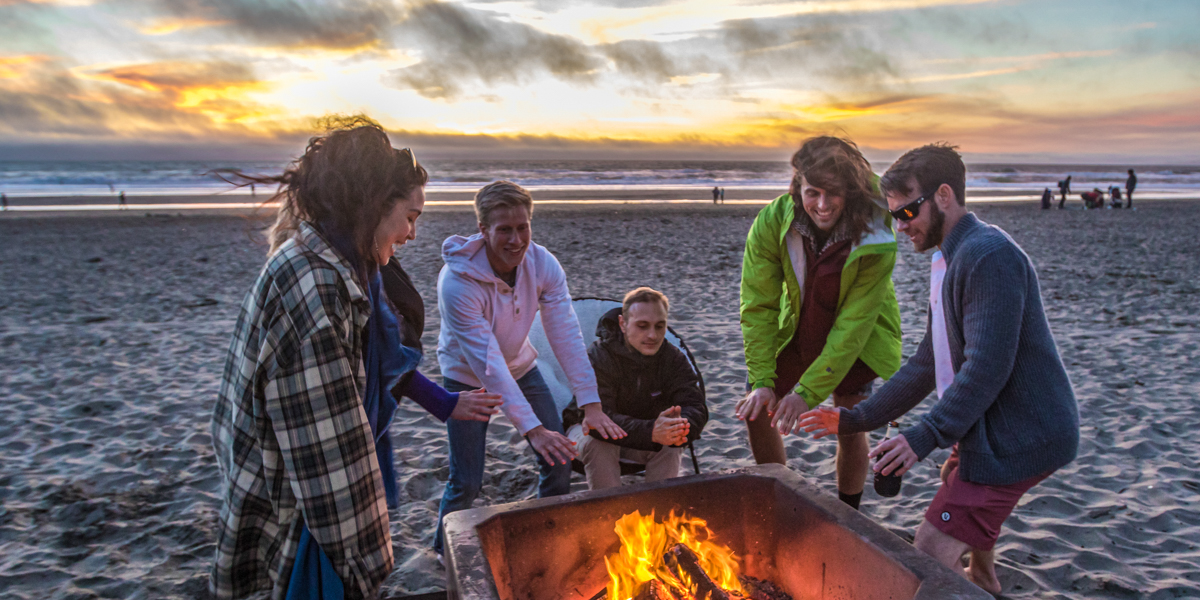In the photograph, a group of six friends, possibly siblings, are gathered around a fire pit on a beach during dusk. The sky is illuminated with hues of orange, hinting at a sunset over the ocean in the background. The cool weather is evident as everyone is wearing jackets and holding their hands over the flames to warm themselves. The fire pit, resembling a large metal container designed for fires, serves as the focal point in the center of the image. In the close foreground, a girl in plaid stands out amidst others clad in solid colors such as blue, green, black, and white. The sandy beach stretches behind them, with the ocean and evening sky framing the scene. Other people can be seen in the distance, adding depth to this cozy yet brisk beach gathering.